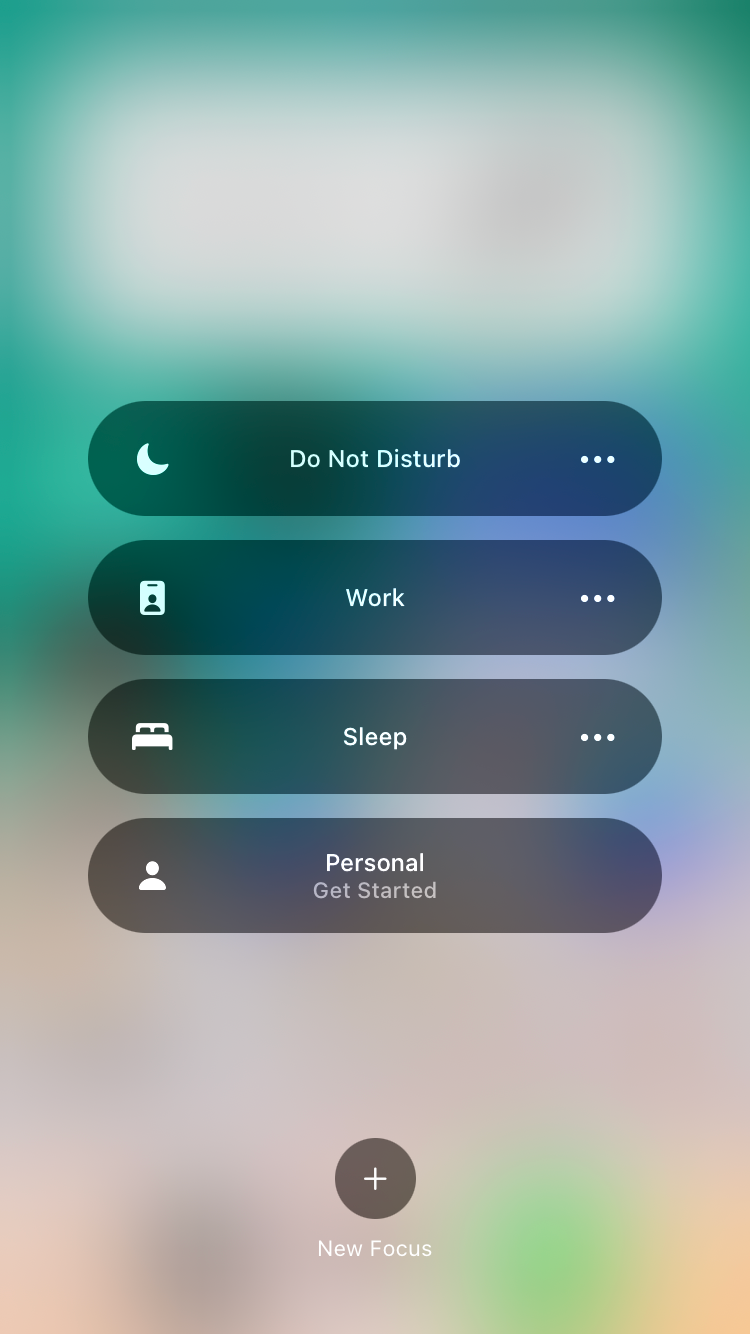This screenshot showcases a device interface with a visually striking, blurred multicolored background featuring hues of teal and purple. Central to the image are four pill-shaped categories displayed in a charcoal gray color.

1. The top category is marked by a white crescent moon icon on the left, labeled "Do Not Disturb" in the center, and includes three horizontal white dots on the right.
2. The second category features a square icon with a head-and-shoulder profile, labeled "Work," also accompanied by three horizontal white dots on the right side.
3. The third category is signified by a double bed icon, with "Sleep" written in the center and the usual three horizontal white dots on the right.
4. The fourth and final category presents another head-and-shoulder profile icon, labeled "Personal," with "Get Started" written below it in lighter gray text.

At the bottom of the screen, there's a circular gray button with a plus sign in its center, labeled "New Focus" in white font beneath it. Additionally, at the top of the screen, a lilac purple bar overlays certain elements, indicating highlighted sections.

The entire interface uses white font within the gray bars, providing a clean contrast except for the "Get Started" text, which appears in a lighter shade of gray against the charcoal pill bar.